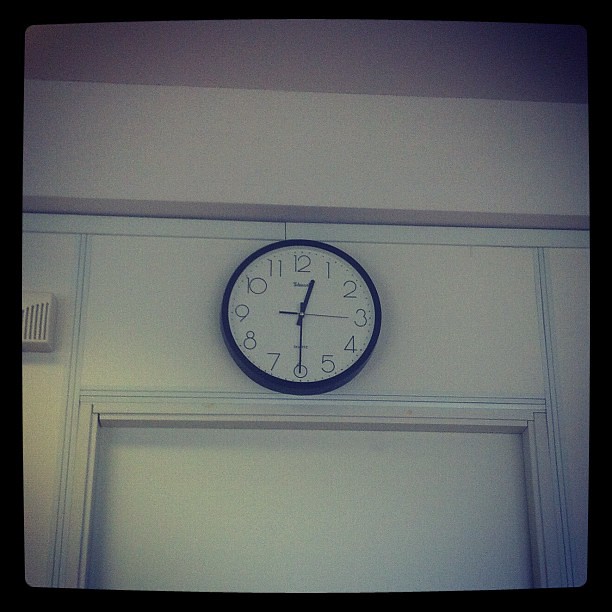In a commercial room, likely part of a conference area within a hotel, a white door with a matching doorframe stands prominently against a wall adorned with white prefab paneling, meticulously joined with white metal channels. Above the door is a classic round clock, its black exterior contrasting sharply with its white face. The clock displays the time as 12:30, with its black hour, minute, and second hands indicating precise timekeeping, the second hand poised at the three. The ceiling in the room is crafted from an off-white or beige drywall, adding a subtle warmth to the otherwise plain decor. Adjacent to the clock, a device resembling a door chime is mounted on the wall, completing the functional aesthetics of the space.